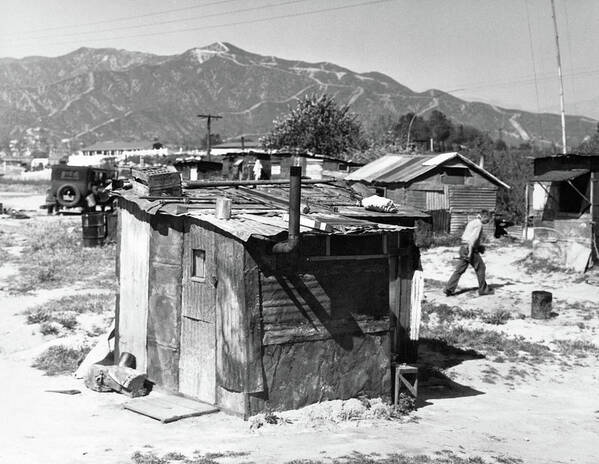The image is an old black-and-white photograph that appears to date back to the 1960s or 70s, depicting a work site with a desolate, sandy terrain and a few patches of grass. Dominating the background is a large, towering mountain range, framed by telephone poles and lines stretching across the top of the photograph. In the foreground, a series of small, square buildings—reminiscent of makeshift shacks—are constructed from a mix of concrete, wood, and metal. Some of these structures have pipes protruding from them, and they seem to lack windows, being boarded up or covered in a dark, weathered material. Scattered across the site are barrels, one of which might be a burn barrel. An old-school car can be seen further back, enhancing the historical atmosphere of the scene. To the right side of the image, a man dressed in dark pants and a long-sleeved, collared shirt is walking, suggesting he might be leaving this work area. The overall setting evokes a sense of rugged, industrial activity against a backdrop of natural grandeur.